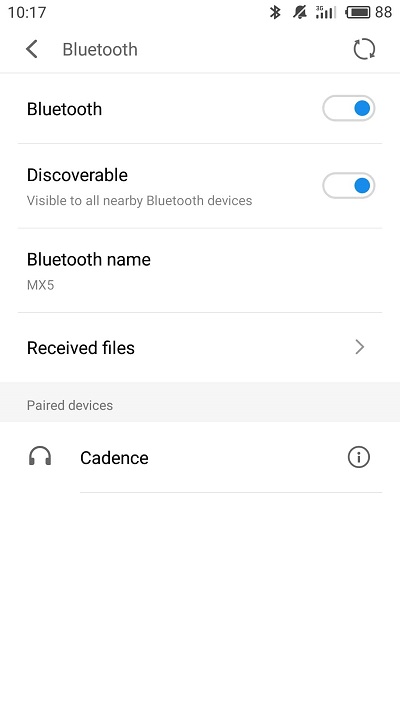This image is a screenshot of a smartphone's Bluetooth settings screen. At the top of the screenshot, the status bar displays the time as 10:17, alongside icons indicating an active Bluetooth connection, a silenced notification bell, full cellular reception with four bars, and a battery life of 88%. Below the status bar, a back arrow icon on the left-hand side indicates navigation options. The title "Bluetooth" is displayed prominently, followed by a secondary heading also labeled "Bluetooth."

The Bluetooth function is toggled on, as indicated by the active slider button. The setting is marked as "Discoverable," making the device visible to all nearby Bluetooth devices. The device's Bluetooth name is listed as "MX5." Further down, there are sections for "Received files" and "Paired devices."

A paired set of headphones, named "cadence," is shown with an accompanying icon of headphones. On the same row, there is a black circle with an information "i" icon, typically used to access additional details about the device. This image is strictly informative and dry, devoid of any photographic elements or representations of people, animals, buildings, plants, vehicles, or other typical photographic subjects. It is a purely functional screenshot, intended to display the Bluetooth settings on the smartphone.